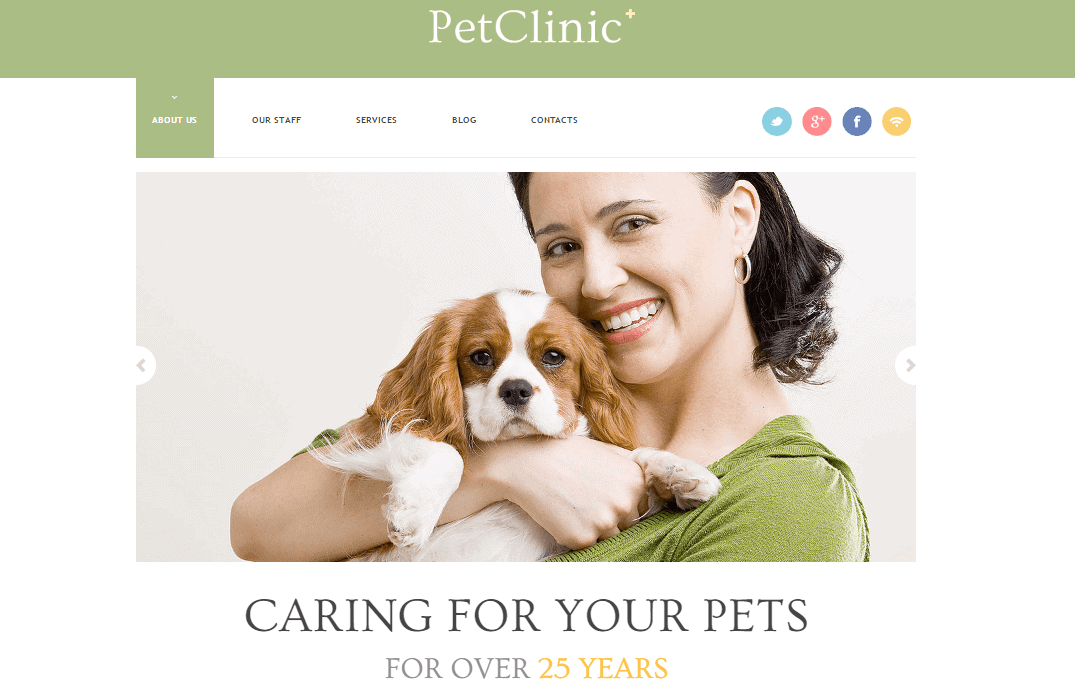The top portion of the image features a banner in an olive green color displaying the text "Pet Clinic." Below this banner are links labeled "About Us," "Our Staff," "Services," "Blog," and "Contacts." To the right of these links are circular icons for social media platforms: Twitter, Google Plus, Facebook, and an orange circle with a Wi-Fi icon.

Beneath the banner, there's a background with a gray hue featuring an image of a woman with black hair. She is holding a dog that has long brown ears, white paws, and a white face. Both the woman and the dog are looking directly at the camera. 

The woman is wearing a green shirt, gold hoop earrings, and has brown eyes with a light complexion. 

Underneath the picture, in large black capital letters, the text reads "CARING FOR YOUR PETS." Directly below this in smaller gray letters is the phrase "for over," followed by "25 YEARS" in gold letters.

The remainder of the image consists of empty space.